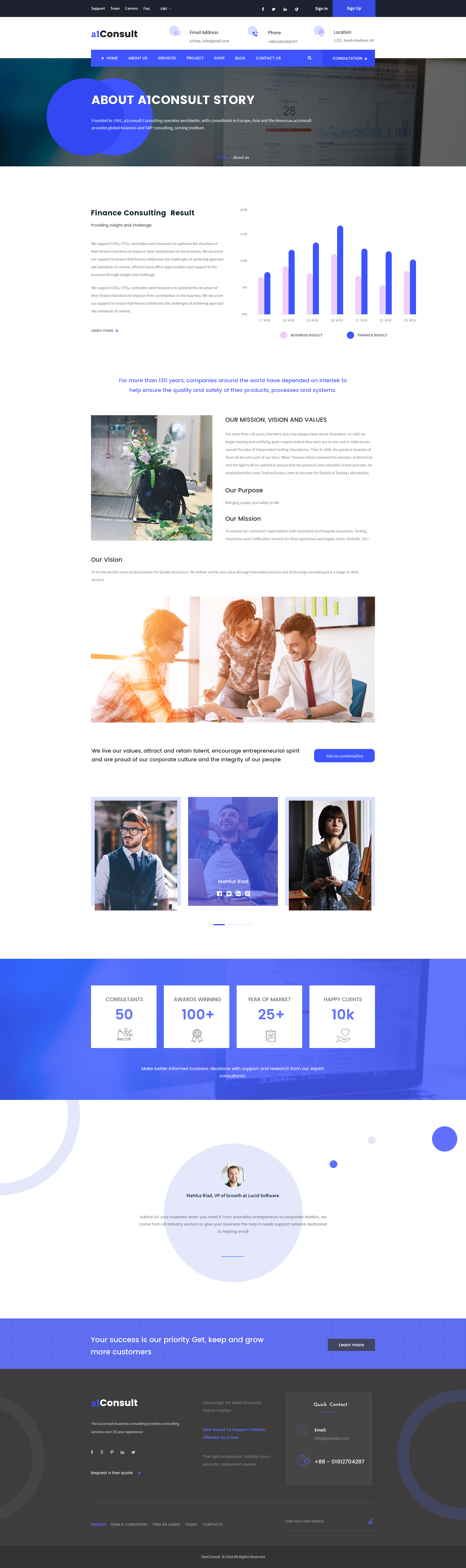The image in question is a vertically oriented rectangle filled with various segments of text and graphical elements. At the top, there's a black bar featuring five clickable items, followed by a black space, another set of four clickable items, a black space, and a singular clickable item in white. Below this is another horizontal bar, this time in blue, with the remaining section being primarily black in color.

The first white space below this sequence contains the text "AI Consult," followed by three distinct groups of text, each separated by additional white spaces. Below these text groups is a black rectangle titled "About AI Consult Story," with a small blue bar positioned above it.

Further down, after a white space, there is a segment of text adjacent to a graph. The graph is rendered in pink and blue. Underneath this graph is more small text, followed by an image of a potted plant.

Directly beneath the plant image is text, and then an image depicting three people working at a table. This image is followed by a row of three squares: the leftmost square shows a man, the middle one is indiscernible, and the rightmost square shows a woman.

Next, there is a blue box containing four information squares displaying the numbers—50, 100+, 25+, and 10k. Below this is an oval-shaped element containing additional information, then a blue box, and finally, a black box, both of which also contain text.